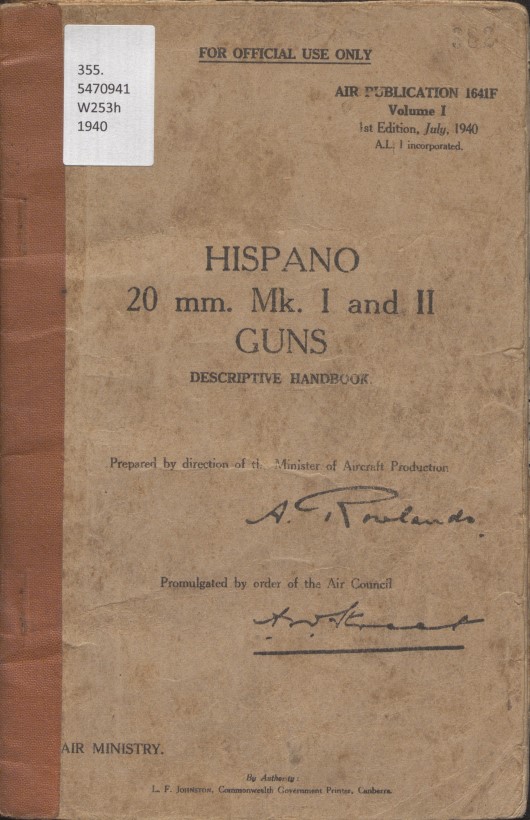This is a detailed photograph of an old and worn manuscript book from a library, identifiable by a sticker labeled with item number 355-547-0491 W233H 1940. The manuscript features a light brown cover with a glued binding, indicating its age and heavy use. At the top of the cover, "For Official Use Only" is prominently stamped, alongside the title "Air Publication 1641F, Volume 1, 1st Edition, July 1940." The book is a descriptive handbook titled "Hispano 20mm MK 1 and 2 Guns," prepared by the direction of the Minister of Aircraft Production. There are signatures on the cover, one of which is A. Rubendy. The overall appearance of the manuscript is very worn and tattered, suggesting extensive handling and use over the years.